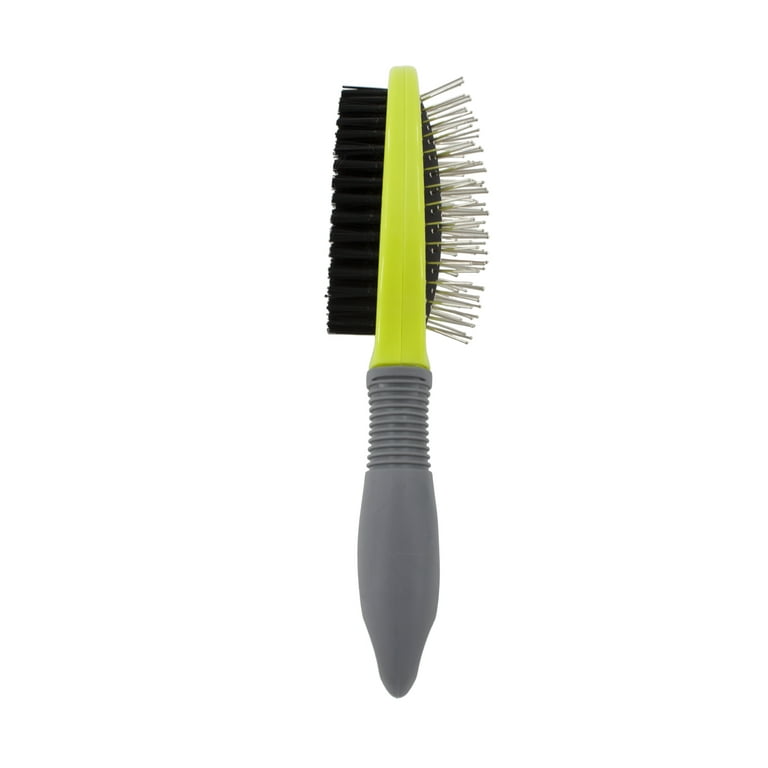This detailed image depicts a dual-sided hairbrush set against a clean, white background, making it the clear focal point. The brush features a primarily gray plastic handle with a smooth grip that narrows to a point at the end. The upper portion of the handle has a distinct ridge leading to a lime green midsection. The brush head is differentiated into two sides: the right side has stiff, wire bristles arranged sparsely on a black cushioned bed, forming a rounded surface. In contrast, the left side is densely packed with soft, uniform black polyester bristles, creating a flat appearance. The detailed textures and dual functionality of the brush are clearly highlighted in this profile view.